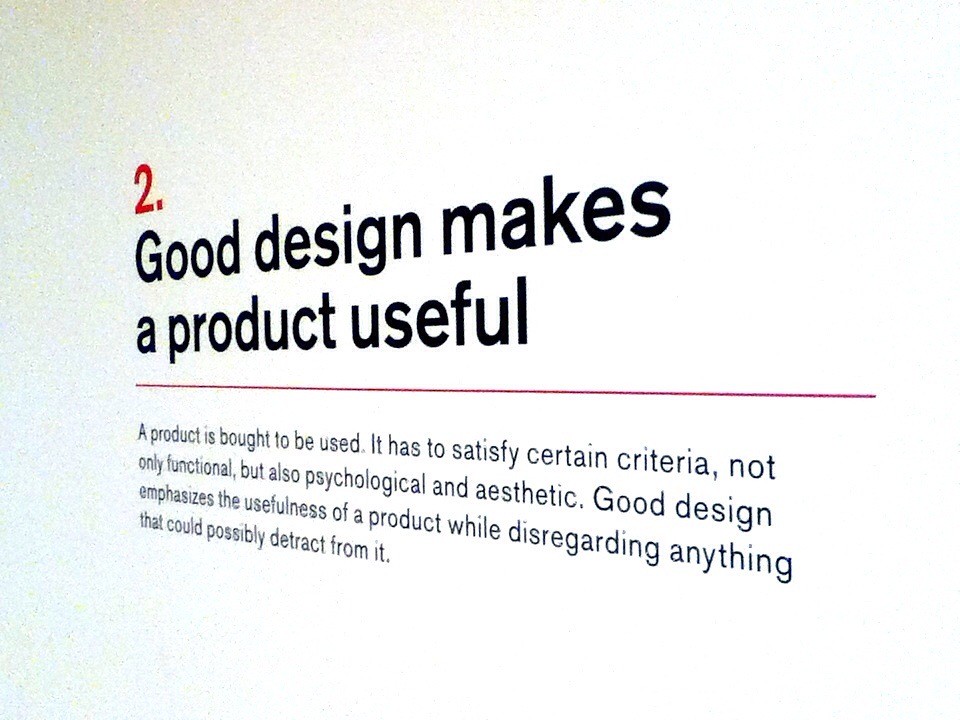The image is a photograph of text that appears to have been taken from a textbook or a sign, viewed from a slight angle originating from the bottom right. The background is primarily white with a noticeable grain, especially towards the top left, giving it a texture akin to film grain. At the center of the image is a prominent red number "2." Directly below this number, in large bold black text, is the phrase "Good design makes a product useful." A thin red horizontal line separates this title from the smaller black text below, which reads, "A product is bought to be used. It has to satisfy certain criteria, not only functional but also psychological and aesthetic. Good design emphasizes the usefulness of a product while disregarding anything that could possibly detract from it." The text is slightly angled, suggesting that the photograph was taken from a perspective that recedes towards the left. The overall image is framed on an off-white background with grain more concentrated at the top left, becoming clearer and smoother towards the bottom and right of the image.